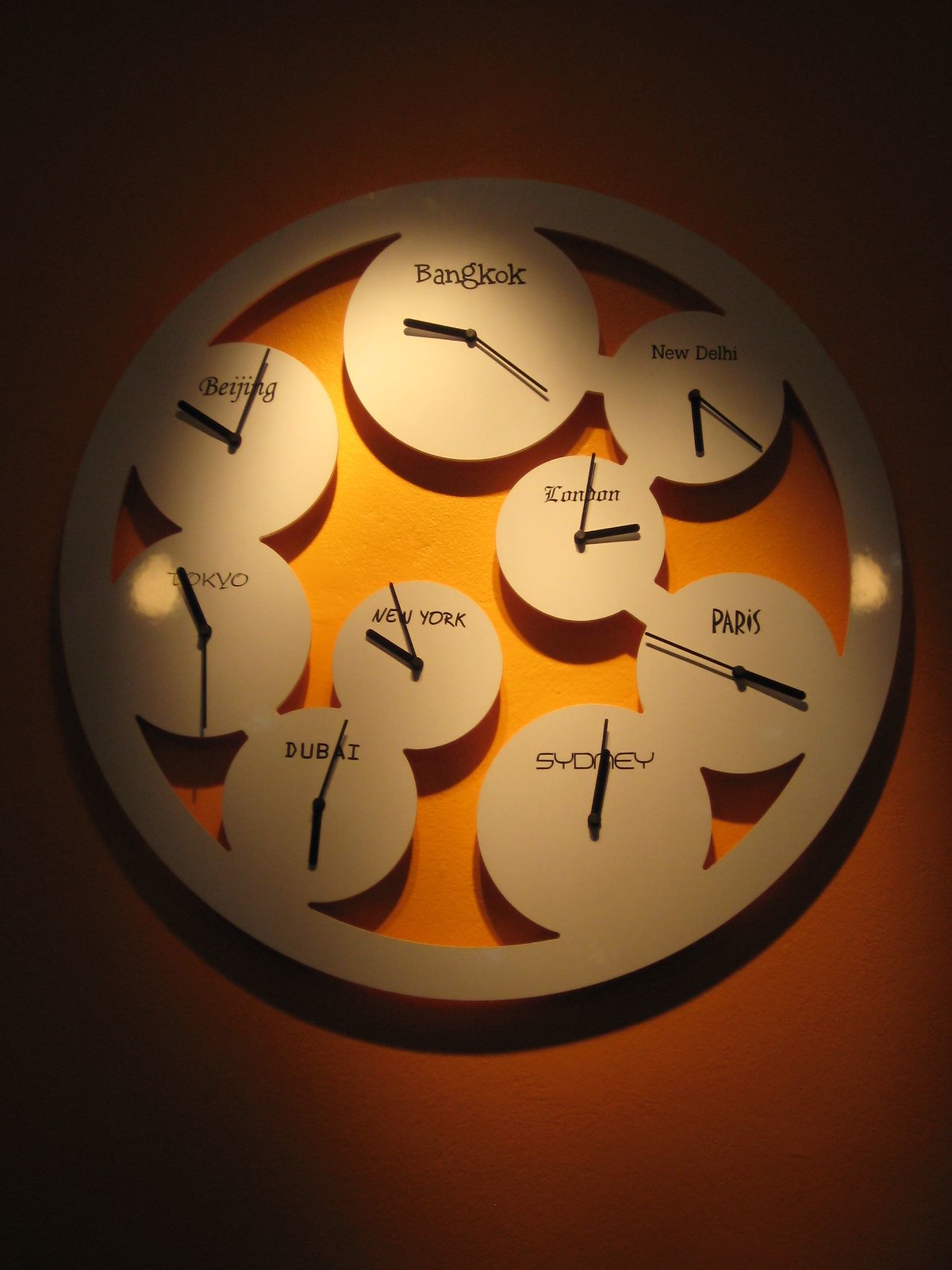This vertical world clock, mounted on an orange wall, features nine smaller clocks encased within a larger, three-dimensional circular frame with a substantial border. Each clock represents a major global city, displaying local times with black minute and hour hands. The layout of the clocks follows a specific arrangement:

- At the top center is Bangkok showing approximately 9:20.
- Positioned to the right of Bangkok is New Delhi.
- Below New Delhi is London.
- Near the 4 o'clock position, you'll find Paris, which is adjacent to the clock for Sydney.
- On the left-hand side at the 7 o'clock position is Dubai, placed just below New York.
- From Dubai, moving towards the 9 o'clock position is Tokyo.
- Directly above Tokyo is Beijing.

The clocks are interconnected by bridge-like connections, guiding the viewer’s eyes smoothly from one clock to the next, embodying a seamless representation of global time zones.